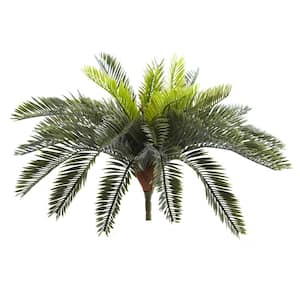This image features a plant set against a white background, likely artificial due to the perfect symmetry of its thick green stem. The plant resembles a fern and has a distinctive structure: the central stem is brown and transitions into a series of leaves that cascade downward in all directions. The leaves vary in color depending on their position; those at the top are a light lime green, while the lower leaves are a deeper, darker green. The leaves at the top are also shorter than the longer ones at the bottom, creating a gradient of hues and lengths that give the plant a lively, feathered appearance.